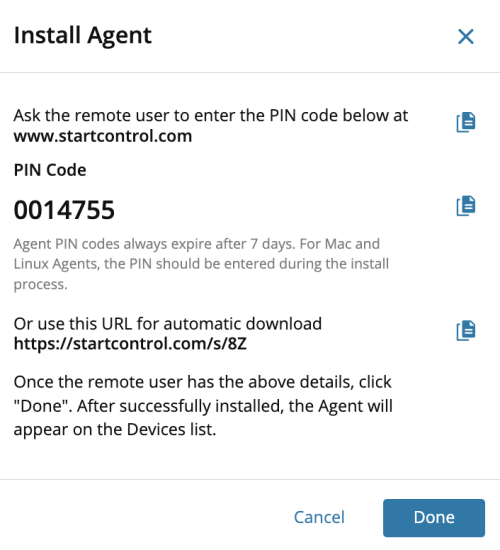The image is a screenshot with a white background and black text. At the top, it reads "Install Agent" with both 'I' and 'A' capitalized. Toward the right, there is a blue 'X' icon. Below this, a thin line separates the header from the content below. The instructions state, "Ask the remote user to enter the PIN code below at www.startcontrol.com". The word 'PIN' is fully capitalized.

Next to this message, there's a blue graphic resembling a piece of paper with a bent top-right corner. Beneath it, the text reads "PIN Code" with 'PIN' fully capitalized and 'Code' with an initial capital 'C'. The specified PIN code is 0014755.

Additional information states that agent PIN codes expire after seven days and highlights that for Mac and Linux agents, the PIN should be entered during the installation process. Further instructions provide a URL for automatic download: "https://startcontrol.com/S/8Z".

Finally, it says, "Once the remote user has the above details, click 'Done'". The word 'Done' is capitalized and in quotation marks. It concludes by indicating that after successful installation, the agent will appear on the devices list.